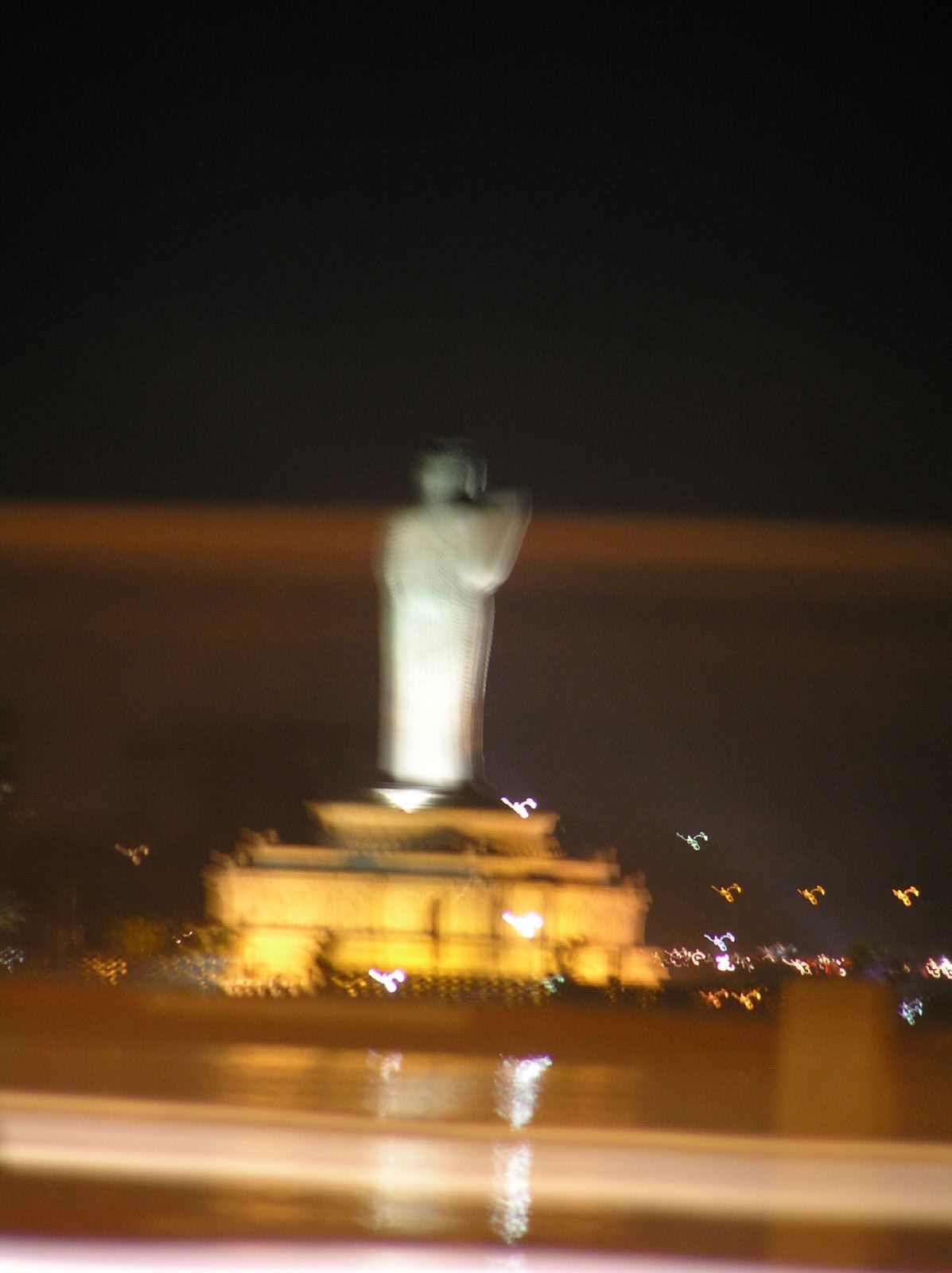Captured through the window of a moving vehicle, this nighttime photograph exhibits a sense of motion and blur. The upper half of the image is enveloped in pitch-black darkness, while the lower half of the sky is tinged with an orangey-brown hue, suggesting the presence of city lights or a distant horizon. Dominating the distant landscape is a large, light green and white statue, reminiscent of the Statue of Liberty, perched atop an expansive whitish-yellow building. Scattered throughout the background are various other lights, adding to the urban atmosphere of the scene.